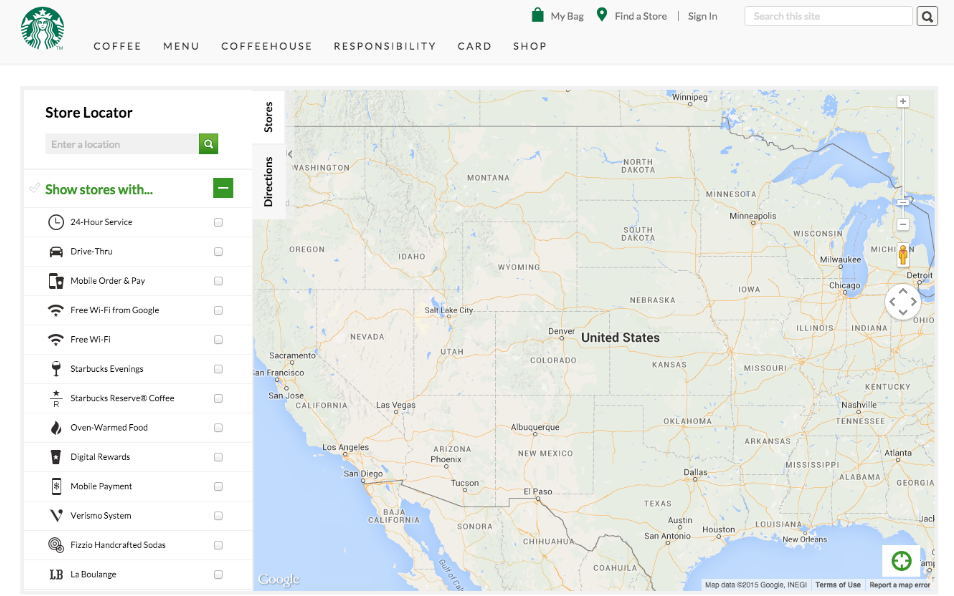The image portrays a detailed map of the United States, prominently featuring the Starbucks logo and elements related to the renowned coffeehouse. The map is overlaid with various interactive features commonly associated with finding Starbucks locations. Key elements include:
 
- A Starbucks logo indicating the prominent branding.
- A coffee menu outlining a variety of beverage options.
- An "Our Responsibility" section possibly highlighting corporate social responsibility initiatives.
- A card for possible loyalty programs or payments.
- A representation of a shop or coffeehouse atmosphere.
- A green shopping bag, symbolizing sustainable or eco-friendly practices.
- A search bar with a magnifying glass icon for finding specific stores.
- Green location markers on the map for identifying Starbucks locations.
- Features for filtering search results based on specific services like 24-hour services, drive-thru, mobile order and pay, and free Wi-Fi provided by Google.
- Various store amenities such as warm food, oven-warm food, digital rewards, mobile payment options, and exclusive Starbucks Reserve coffee options.
- Additional icons and symbols for handcrafted beverages, soda options, and a lounge area named "La View Lounge."

The overall layout seems to be an interactive and user-friendly interface designed for efficiently locating and exploring Starbucks stores across the United States, showcasing the brand's commitment to wide-ranging services and consumer convenience.